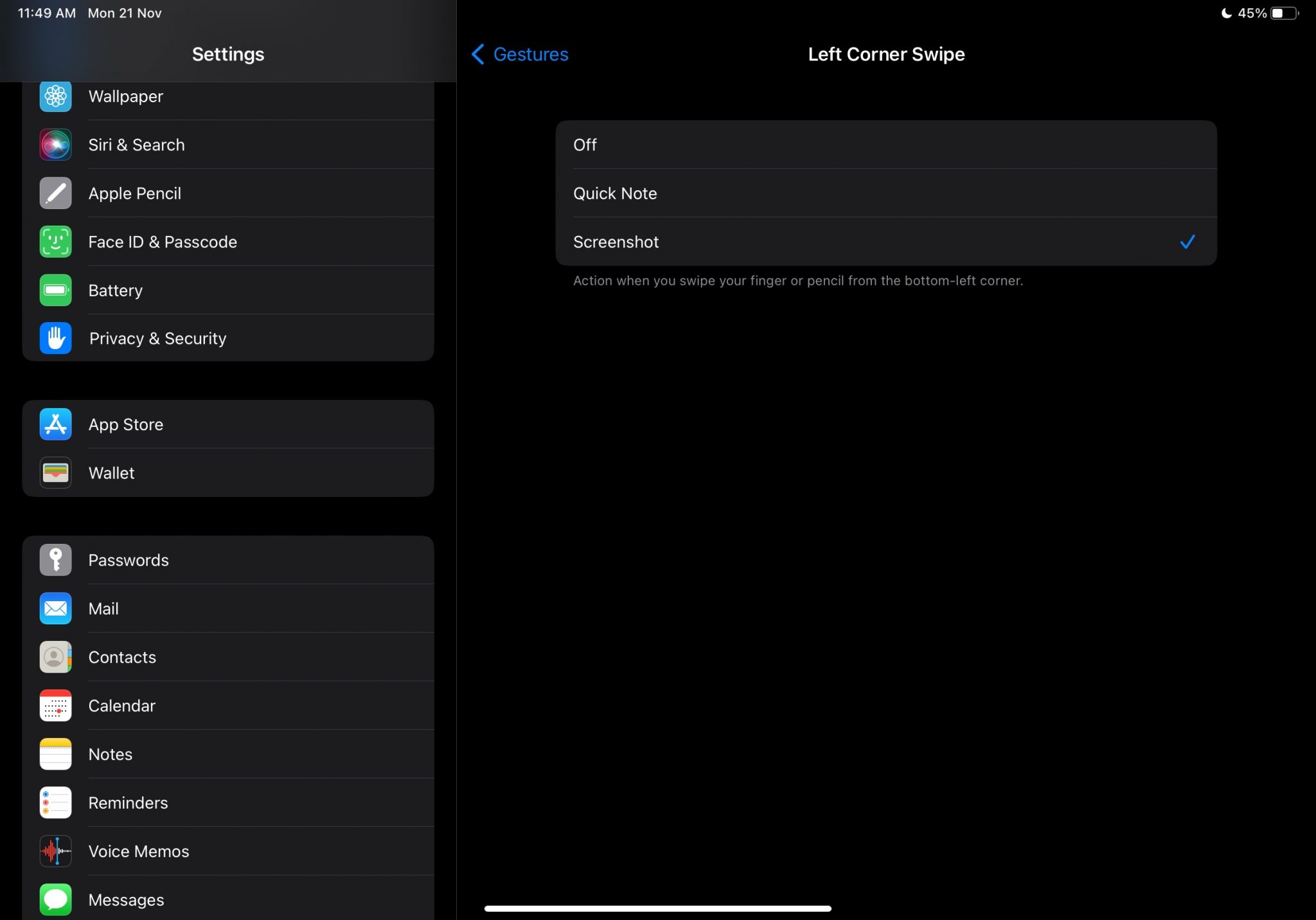This is a screenshot of an iPad settings page captured at 11:49 a.m. on Monday, 21 November. The screen has a black background with white text. In the upper left-hand corner, the time is displayed, while the upper right-hand corner shows a half-moon icon and a battery icon indicating 45% battery life.

The main focus of the screen is a section titled "Gestures" in blue text. Below this heading, in white text, it says "Left Corner Swipe." Under this, there are three options listed within a rectangular selection box: Off, Quick Note, and Screenshot. "Screenshot" is selected, marked by a blue checkmark.

Running along the left side of the page is a vertical menu displaying various settings, each accompanied by a colorful icon, predominantly in shades of blue or green. The settings listed from top to bottom are: Wallpaper, Siri and Search, Apple Pencil, Face ID and Passcode, Battery, Privacy and Security, App Store, and Wallet.